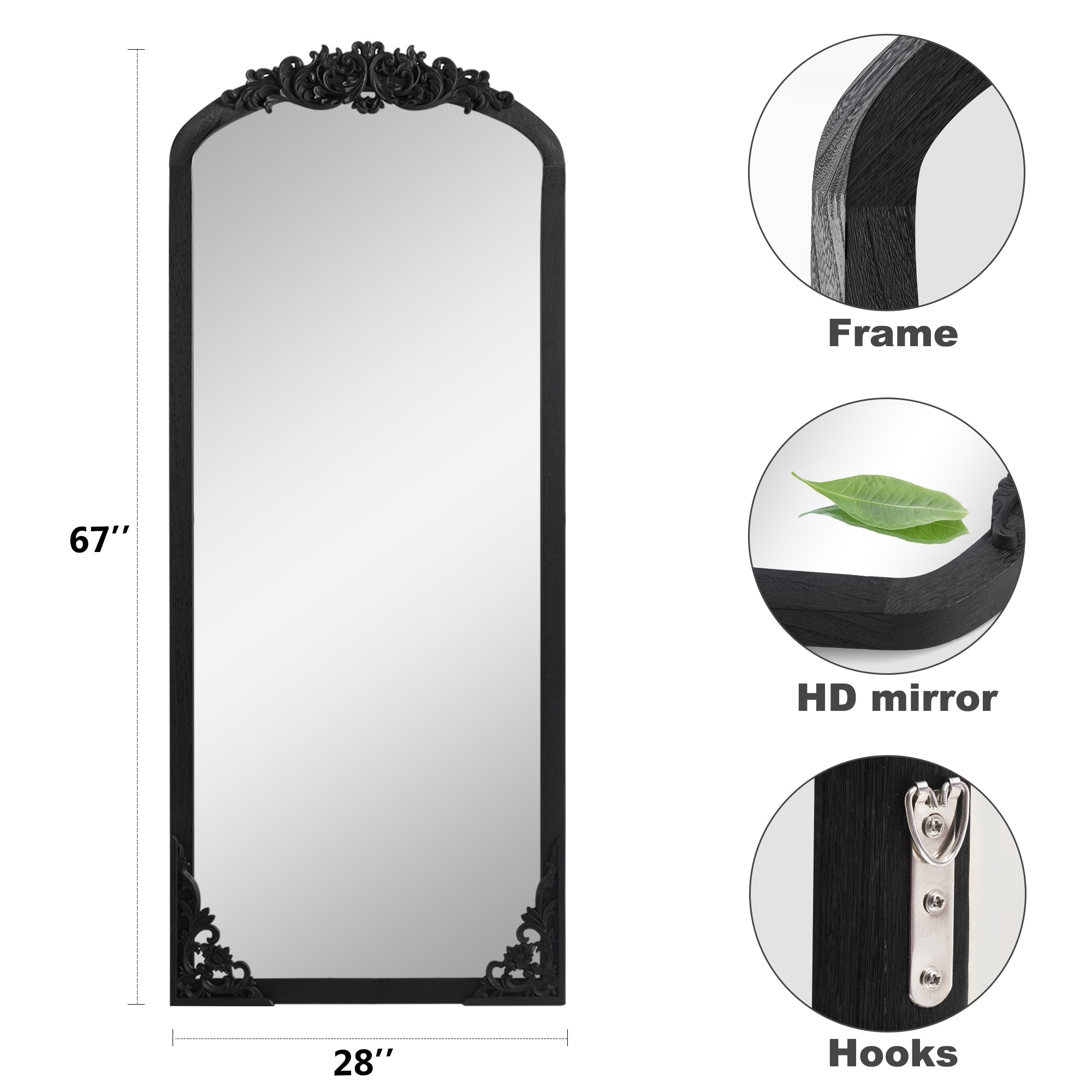The image is a marketing-style photograph of a tall, full-length mirror, isolated on a white background, accompanied by three circular close-ups illustrating detailed features. The mirror, measuring 28 inches wide by 67 inches tall, has a black painted, ornately carved wooden frame. The top of the mirror features a low-degree arch adorned with a vine-like leaf design, while the bottom corners are squared with decorative inlaid carvings. The left side of the image includes dimension lines for height and width. On the right, three circles highlight specific details: the first displays a close-up of the frame's upper curve labeled "FRAME," showcasing the intricate woodworking; the second, labeled "HD mirror," emphasizes the high-definition clarity of the reflective surface; and the third, labeled "HOOKS," shows the metal attachments on the back of the frame for secure wall mounting. There is a green leaf reflected in the mirror, demonstrating its excellent reflective quality.